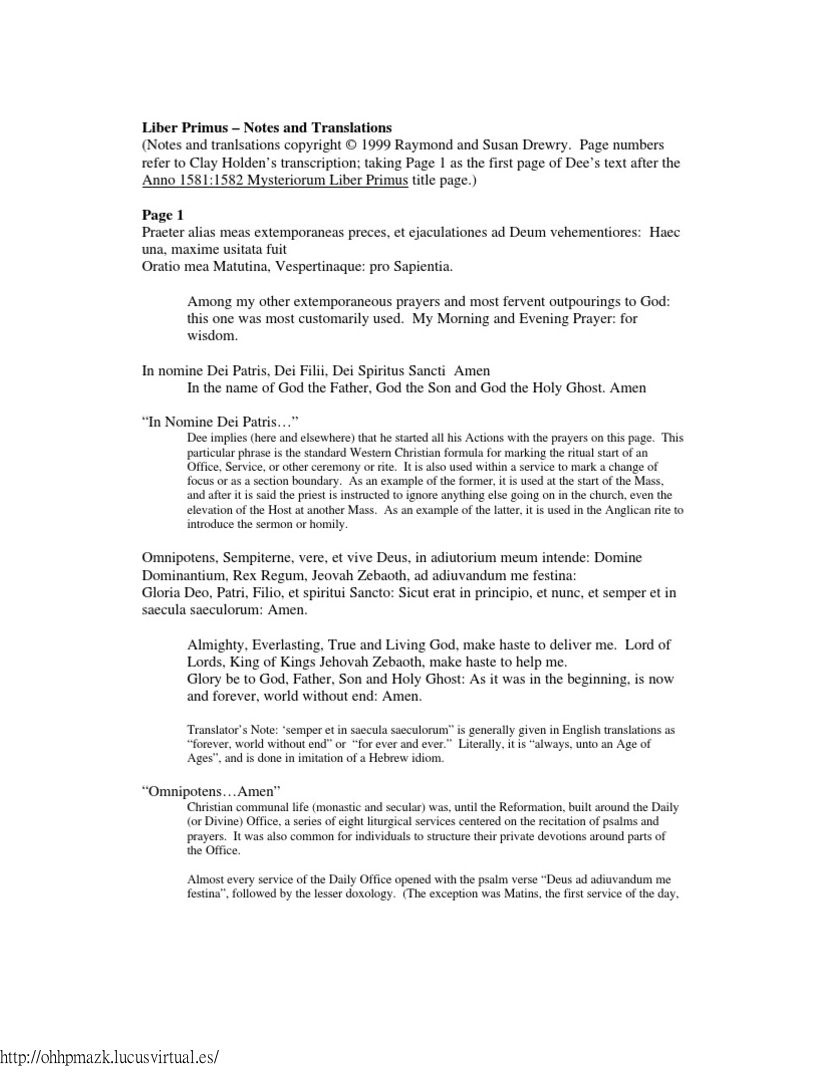The image displays a vertically aligned rectangular document with text against a solid white background, without a border. It consists of several paragraphs. At the top, in bold, it reads "Libre Primus - Notes and Translations." Following this are three lines of text. There is another bold heading labeled "Page 1," under which there are three more lines of text. Most of the content is left-aligned, except for a few centered lines under the headings. The document includes religious phrases such as "Almighty, Everlasting, True and Living God, make haste to deliver me, Lord of Lords, King of Kings, Jehovah, Zeboth, make haste to help me, Glory be to God, Father, Son and Holy Ghost, as it was in the beginning, is now and forever, world without end, Amen," suggesting it's a collection of prayers.

There are also several Latin phrases, including "Omnipotens sempiterne verus et vivus Deus, ad adiuvandum me festina," and English translations interspersed with explanations indicating its use in Christian liturgical tradition. At the bottom left corner, the source is cited as "http://OHH-PMAZK.LucasVirtual.es/." This detailed document appears to be an excerpt or transcription of religious texts, perhaps used in both communal and private devotions, marked by traditional prayers and liturgical notes.